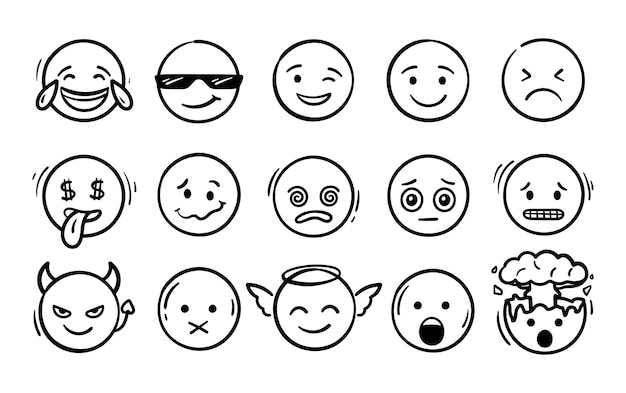The image features a white backdrop with 15 black-and-white emoji-style faces arranged in a grid of three rows and five columns. Each circular face displays a distinct expression. In the top row, from left to right, there is a grinning face with tears of joy, a half-smiling face wearing black sunglasses, a winking and smiling face, a regular smiley face, and a face with arrow-like eyes pointing inward and a downturned mouth. The middle row begins with a face showing money signs for eyes and a tongue sticking out, followed by one with a rueful expression marked by an upside-down eyebrow and a squiggled smile. Next is a face with dizzy spirals for eyes and a frown, another with large pupils and a neutral expression, and finally, a concerned face with gritted teeth and lines indicating worry. The bottom row starts with a devilish face with horns, followed by a face with an X for a mouth, then an angelic face with a halo and wings, a face with wide open eyes and mouth, and lastly, a face that's seemingly blown its top, with a cloud or explosion emerging from a cracked skull.